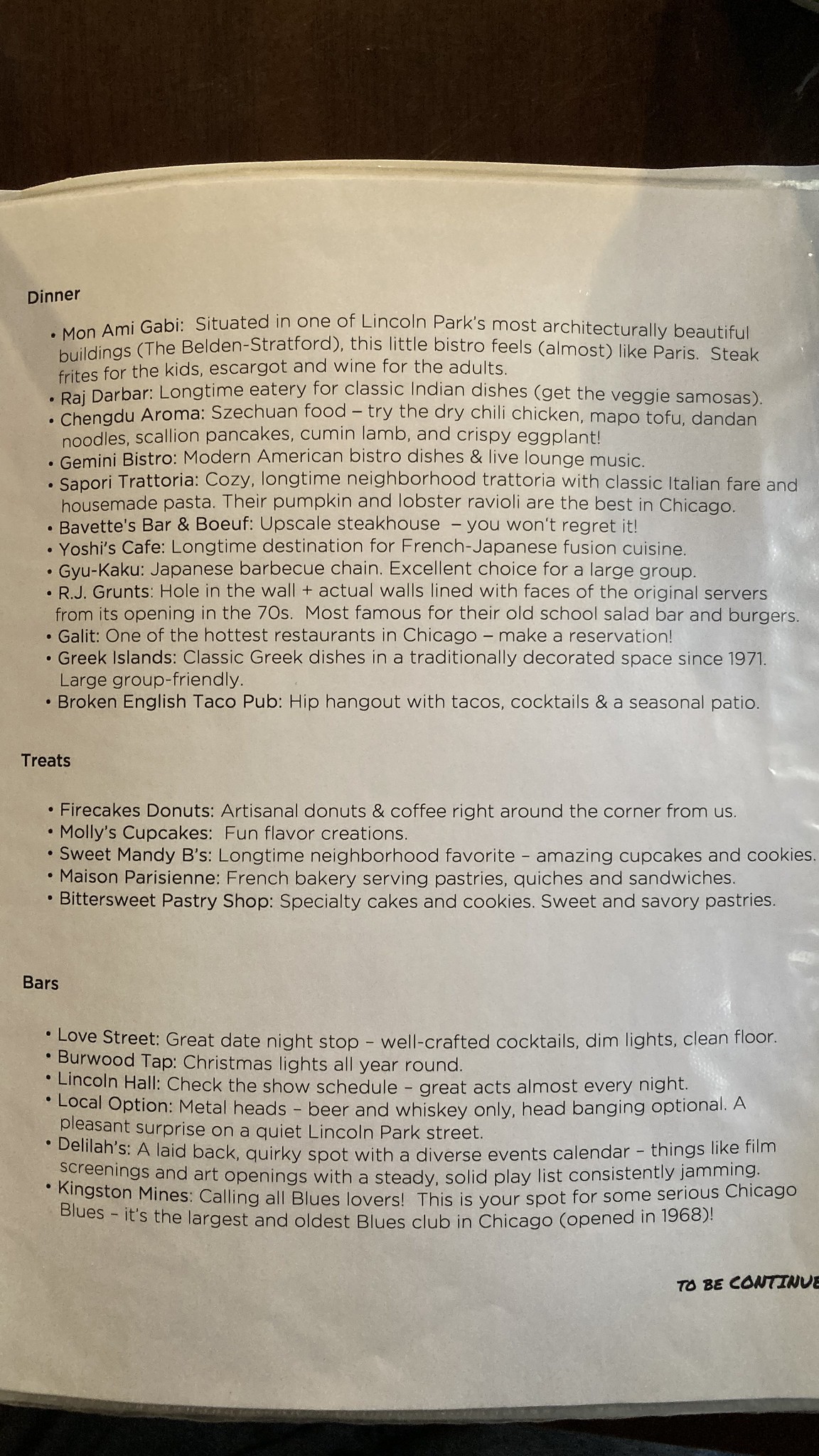This image, likely extracted from a tourist guide provided by a hotel, prominently features dining recommendations in Chicago. The section begins with the word "Dinner" and lists several notable restaurants:

1. **Mon Ami Gabi**: Nestled in one of Lincoln Park's most architecturally stunning buildings, this charming bistro evokes the essence of Paris. It offers a variety of dishes, including steak frites for children and escargot accompanied by wine for adults.

2. **Raj Darbar**: A longstanding favorite for authentic Indian cuisine, this restaurant is known for its classic dishes. The veggie samosas come highly recommended.

3. **Chingu Aroma**: Specializing in Shezong food, this restaurant offers a variety of flavorful options such as dry chili chicken, Mapo tofu, dandan noodles, scallion pancakes, cumin lamb, and crispy eggplant.

4. **Gemini Bistro**: This spot offers modern American bistro dishes, making it perfect for any occasion. Guests can also enjoy live lounge music while dining.

5. **Sampori Trattoria**: A cozy, long-established neighborhood trattoria, it serves traditional Italian cuisine with house-made pasta. The pumpkin and lobster ravioli at this restaurant are touted as the best in Chicago.

6. **Bavette's Bar and Booth**: This upscale steakhouse promises an unforgettable dining experience.

Beneath these recommendations, the guide includes a section labeled "Treats" featuring dessert spots such as Fire Cakes Donuts, Molly's Cupcakes, Sweet Mandy B's, Maison Parisien, and Bittersweet Pastry Shop.

The final section is dedicated to bars and includes recommendations for Love Street, Burwood Tap, Lincoln Hall, Local Option, Delilah’s, and Kingston Mines. The bottom right-hand corner of the page teases a continuation, reinforcing that this is part of a comprehensive guide for tourists exploring Chicago.